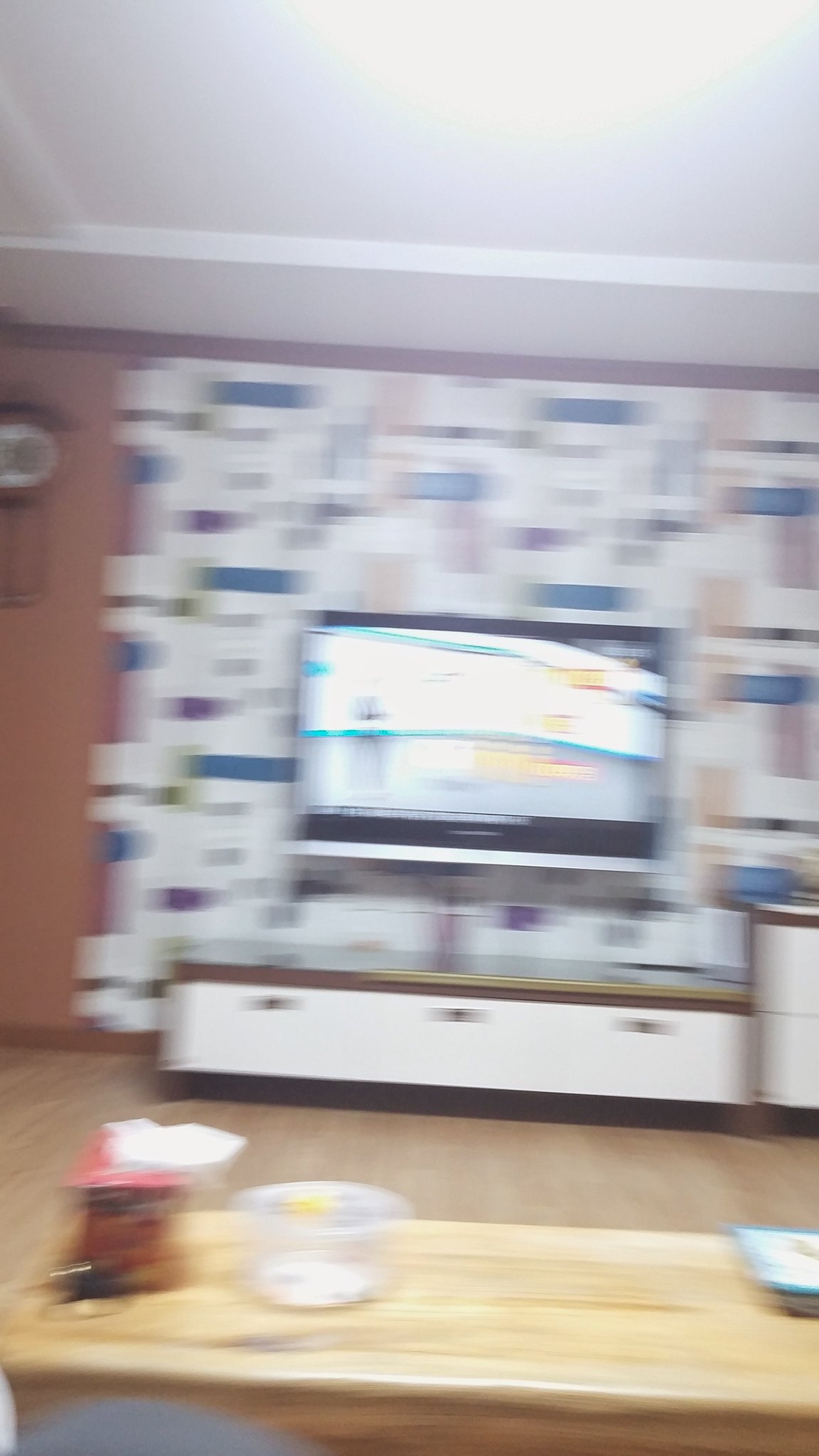This is a color photograph characterized by significant blurriness and lack of focus. At the very bottom of the image, the surface of a desk is discernible, made of light hardwood resembling untreated plywood. Placed on this desk, there appears to be a clear glass coffee mug or cup. Slightly above the desk, a portion of the floor is visible, constructed from a darker-shaded hardwood. The opposite wall, visible in the background, features elaborate decorations comprising geometric shapes in blue and darker gray hues set against a white backdrop. Additionally, a large flat-screen television is mounted on this wall, displaying an indistinct image predominantly in shades of white and blue.